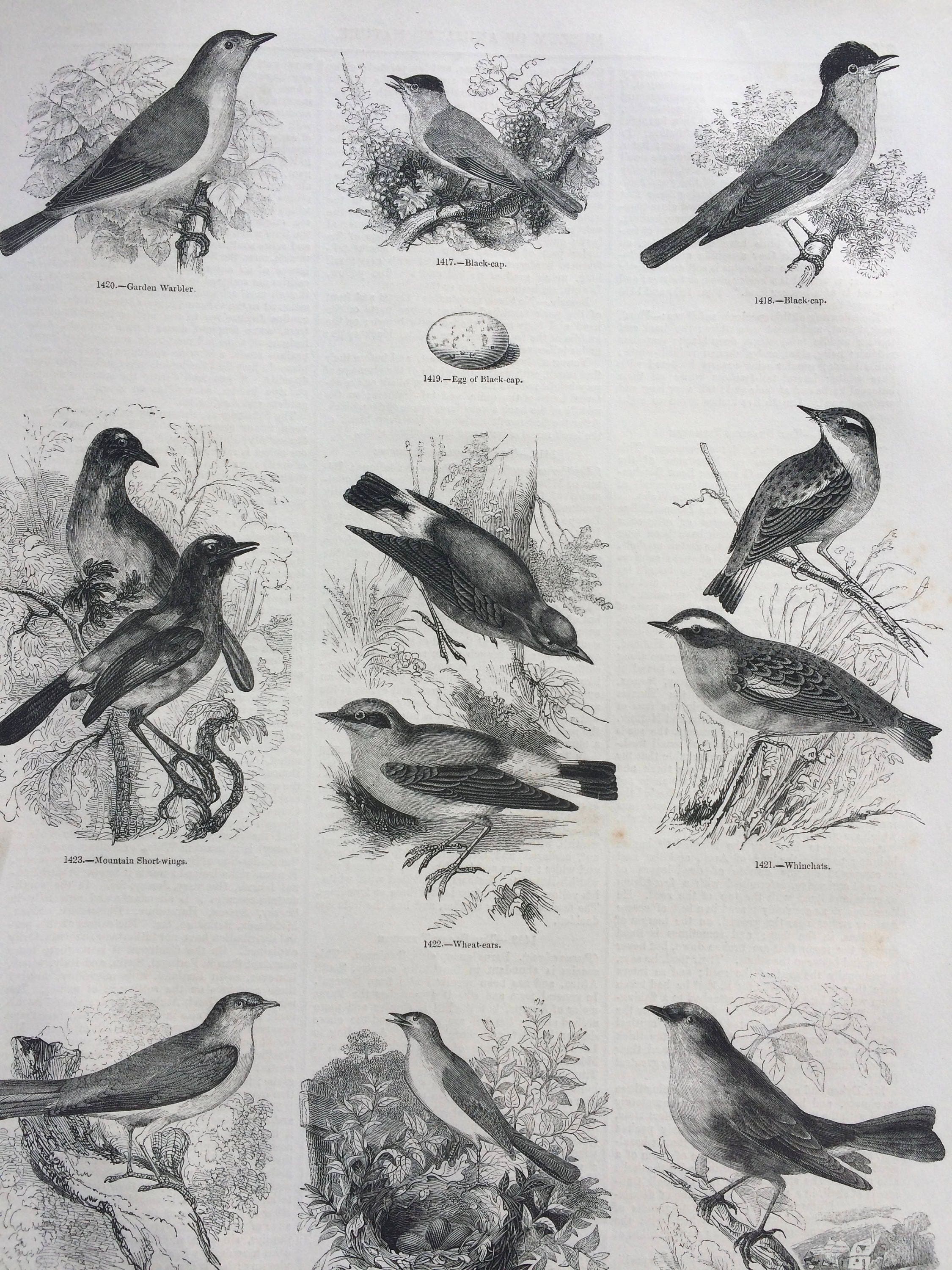The image depicts a page from an old bird identification guide, featuring meticulously drawn black and white illustrations of various small bird species. Each of the approximately nine birds is detailed with short beaks and predominantly perched on branches, amidst a backdrop of foliage. Beneath each bird's image, small black text provides the name of the species, such as garden warbler, black cap, mountain shortwings, wheat ears, and winchats. In the center of the layout is a detailed drawing of a speckled bird egg labeled "egg of black cap." A notable scene includes a bird at the middle bottom of the page, which is standing on a nest with its beak slightly open. The paper has a pale brown or grayish tint, enhancing the vintage feel of the illustrations.